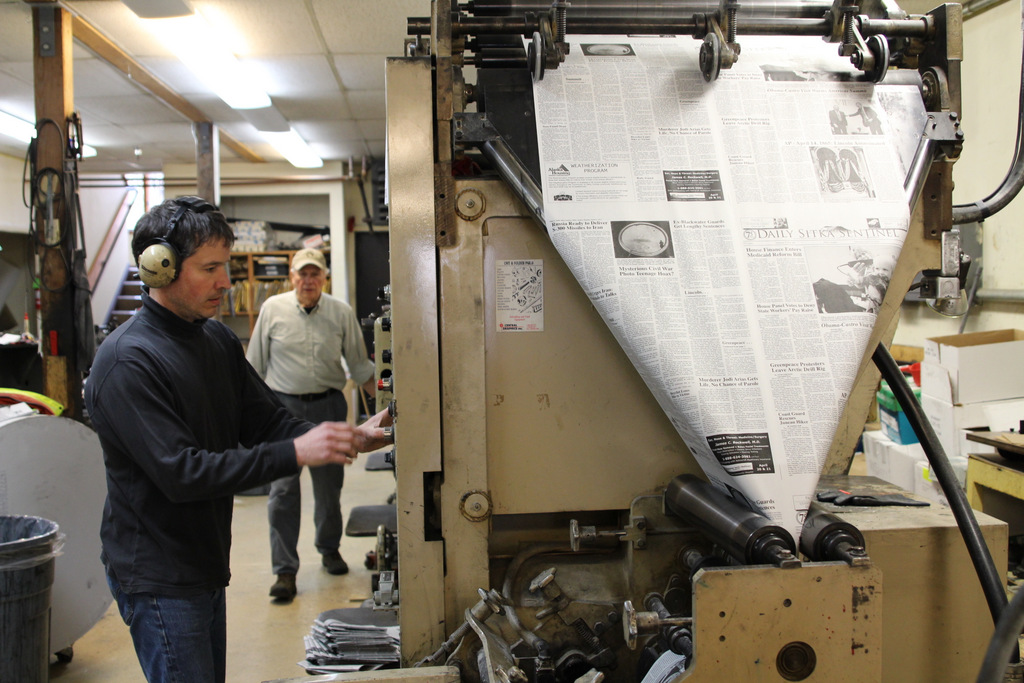The color photograph captures a bustling newspaper printing press facility, possibly situated on the ground floor or in a basement-like setting, as suggested by the lack of windows and the presence of a staircase with a banister leading to another floor. The room is illuminated by fluorescent lighting attached to a drop ceiling, casting a somewhat beige and dingy tan ambiance over the space.

Dominating the scene is a large, beige-colored metal printing press, approximately eight to ten feet high, positioned centrally and extending towards the right side of the image. Newspaper newsprint is seen emerging from the press, running through rollers that keep it flat. There are tubes feeding into this massive machine, which appears to fold the newspapers. 

In the foreground, a young operator with brown hair, wearing ear protection, a black mock turtleneck, and dark blue denim jeans, is meticulously adjusting some dials or buttons on the machine. His focused stance reflects the meticulous nature of his work. Just behind him, an older man dressed in a long green button-down shirt, dark gray pants, and a beige ball cap, is walking towards the younger operator.

The background reveals a built-in wooden shelving unit filled with various supplies, hinting at the operational nature of the facility. Visible to the left, parts of a large gray industrial trash can with a clear plastic liner can be seen, emphasizing the work environment's practical setup. A support beam, possibly adorned with aprons or cords, stands out with a hint of red that may indicate the presence of a fire extinguisher, adding to the safety measures in place.

Overall, the image vividly encapsulates the industrious atmosphere of a newspaper printing press, characterized by its mechanical intricacies and the focused activities of its workers.